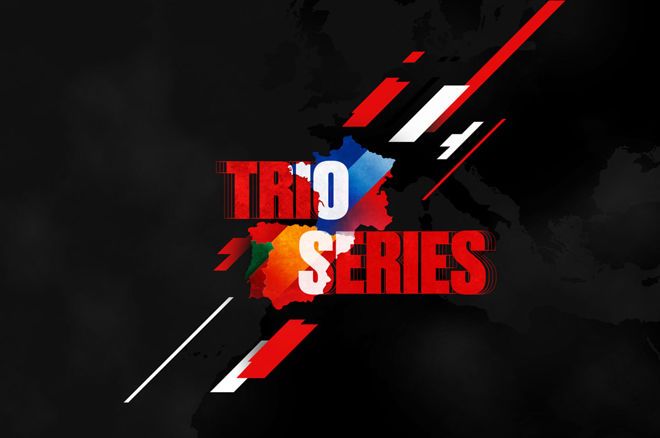The image features a black and cloudy background with a faint silhouette of Europe, extending towards the Middle East. At the center of the image, in a slightly shifted and layered arrangement, are the words "TRIO SERIES." The word "TRIO" appears in red with the 'O' in white, and "SERIES" is primarily in red with a white 'S.' These words create a powerful visual contrast against the dark backdrop.

Superimposed over the countries of Portugal, Spain, and France are their respective flag colors. Portugal is represented with red and green hues, Spain with red and yellow, and France with blue, white, and red—though the white in France merges slightly into a sky blue. These colors are blended into the silhouette of their countries, forming an abstract, flag-like display.

Below the central text, diagonal lines in red, white, and blue extend from the middle left to the middle top, adding texture and visual complexity to the composition. These lines, along with the superimposed national colors, suggest a dynamic and competitive interaction between the countries.